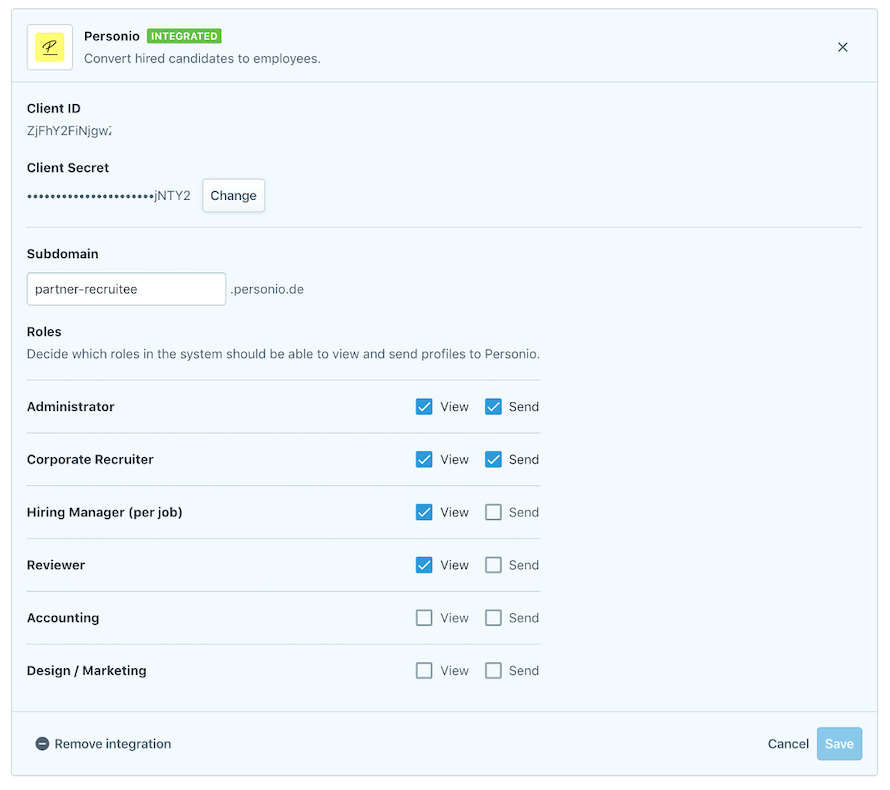The image appears to be a screenshot of a configuration menu from a web page. The background is a very light grayish-blue color, nearly white. At the top left corner, there is a white square containing a smaller yellow square, which features a black cursive "P" in the middle. To the right of this logo, the word "Personia" is displayed in black font. Adjacent to "Personia," there is a small green rectangle with the word "Integrated" written in white font. Beneath this, it reads "Convert Hired Candidates to Employees."

In the upper right corner of the menu, there is a small "X" for closing the menu. Below the header, bold black text labels "Client ID," followed by the ID number "ZJFHY2FINJGW." Next to it is a semicolon, and underneath, labeled "Client Secret," are several asterisks followed by the text "JNTY2." Next to this, there's a small white square button with the word "Change" in black font.

Further down, the word "Subdomain" appears, accompanying a field for input, which currently shows "Partner-Recruiter.personia.de." At the bottom of the menu, there is a section labeled "Roles," with instructions to decide which roles in the system should be able to view and send profiles to Personia.